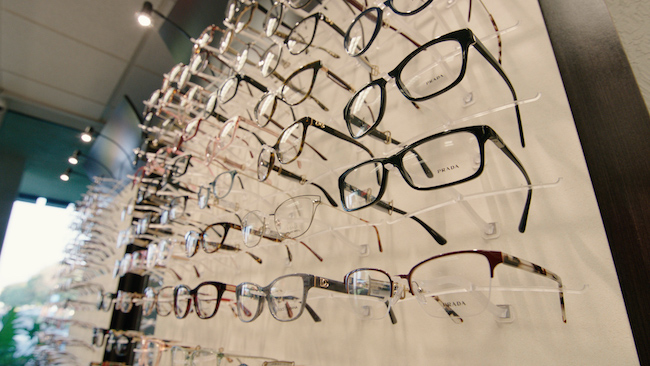The photograph, taken inside an eyeglass store or optometrist's office, captures a stylized display of eyeglass frames from a bottom-right angle, providing a view of numerous rows extending to the ceiling and horizontally to the left. The white background, highlighted by black mortar, showcases clear acrylic hooks supporting an array of eyeglasses with varying styles and colors. The collection includes simple wireframes, masculine black frames, trendy tortoiseshell patterns, gender-neutral gray frames, and even some with pink trims. Many frames bear the Prada logo and are all fitted with clear lenses. Overhead, spotlight lighting accentuates the display, casting reflections off the lenses and emphasizing the meticulously arranged frames. In the background, the ceiling transitions from tan to green, and a window on the far left allows natural light to pour in, with additional exterior views visible through a blurred section. The image's perspective and lighting give a comprehensive yet artistic representation of the vast selection of eyeglasses available.